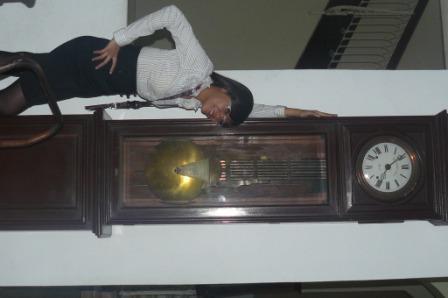A large, elegant grandfather clock with a wooden frame and a prominent, gold-colored pendulum occupies the center of the image. The clock features a white face with Roman numerals. The photograph, taken indoors, is incorrectly oriented in landscape mode and needs to be rotated 90 degrees counterclockwise to view it properly in portrait mode. Standing to the left of the clock is a professional-looking woman with black hair, smiling. She is dressed in a white button-down shirt with dark stripes, tucked into a dark navy pencil skirt that ends around her thigh, complete with dark tights. She wears a lanyard around her neck. Her left arm is raised, palm flat against the side of the grandfather clock, while her right hand rests below her hip. The top and bottom of the clock are slightly cut off from the frame, emphasizing its size, which is approximately twice the height of the woman. The backdrop is a plain white wall, highlighting the clock and the woman's formal attire, suggesting a professional setting, perhaps related to the clock's restoration.